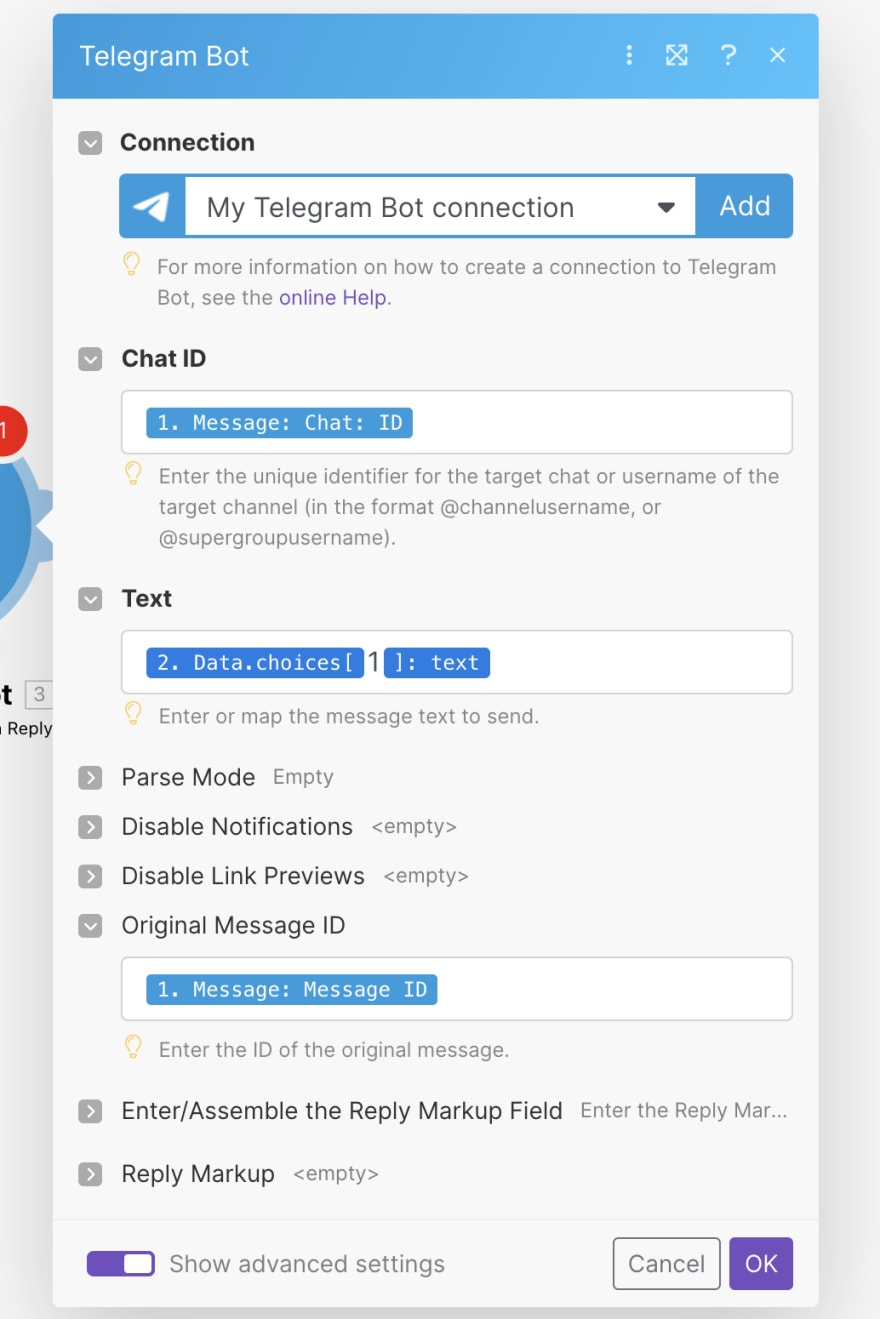The image depicts a website interface layered over another page, evident from the blue background and a red circle visible on the left side. The header at the top is labeled "Telegram Bot" in blue text. On the right side of the page, there are icons and a section that reads "Connection," marked by a gray check box. The interface includes various fields related to the bot's configuration:

- "My Telegram Bot Connection" with an adjacent add button.
- "Chat ID," with text shaded in blue and a gray checked box beside it.
- "Text," also marked by a gray checked box and containing shaded text in blue.
- "Parse Mode," which is empty.
- "Disable Notifications," which is empty.
- "Disable Link Previews," which is empty.
- "Original Message ID," with a bar shaded in blue containing a message.

Down the left side, the boxes are predominantly gray and feature either arrows or check marks. Below these options, there's a section to "Enter and assemble the reply markup field," which is currently empty.

At the bottom of the interface, a "Show Advanced Settings" option is activated, indicated by its purple color. Adjacent to these settings are two buttons: a "Cancel" button and an "OK" button, which is also purple, situated at the right bottom corner.